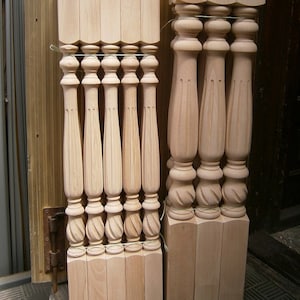The image depicts eight intricately hand-carved wooden spindles, likely intended for use in staircase railings or possibly as bedposts. These plain, untreated spindles, arranged in front of a doorway with a visible hinge at the lower left, show a natural variation in wood tones, ranging from lighter to darker shades. Five narrower spindles are clustered together on the left, while three wider and slightly taller spindles are grouped on the right. Each spindle features a design incorporating three central circles, an element resembling a baseball bat, and additional circular patterns below. Both ends of the spindles are capped with wooden blocks. The background suggests an indoor setting, possibly a workshop, accentuated by the wooden surfaces and a door lock visible on the floor.